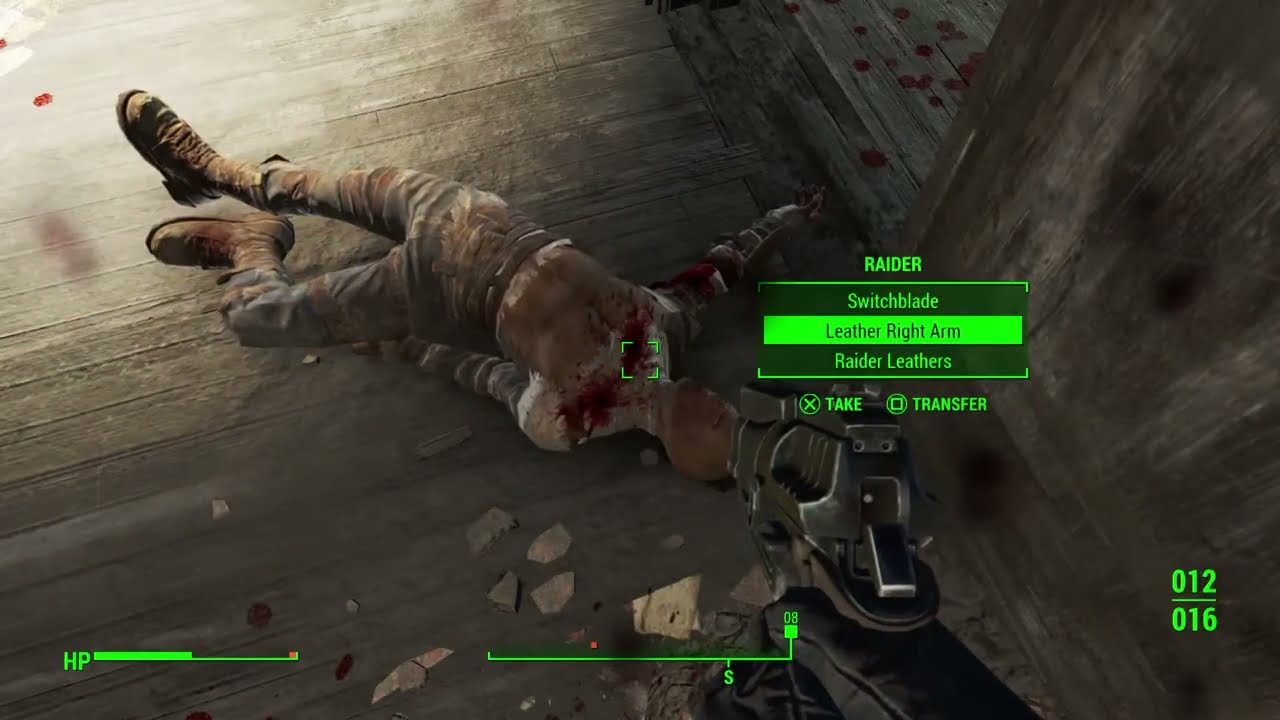The image is a still from a first-person shooter video game, depicting a worn and crumbling facility with gray rubble and light red bricks scattered around a degrading floor and ceiling. In the foreground, a pair of gloved hands holding a silver handgun points at a large, curved mural on a cracked stone wall ahead. The mural features a detailed, animated scene starting from the left with a large military ship and military-style planes soaring above. Centered on the wall, there are three army soldiers dressed in green camouflage, with one wielding a bayonet and the others holding machine guns, all set against a backdrop of the American flag and a fiery explosion. To the right of the soldiers, the mural transitions to a futuristic off-world setting, displaying an astronaut near a lunar base, under a bluish dome. Green numbers "008" and "032" are displayed at the bottom right, and on the far left of the screen, "HP" is shown with a three-quarters full green health bar, suggesting the game’s HUD elements.